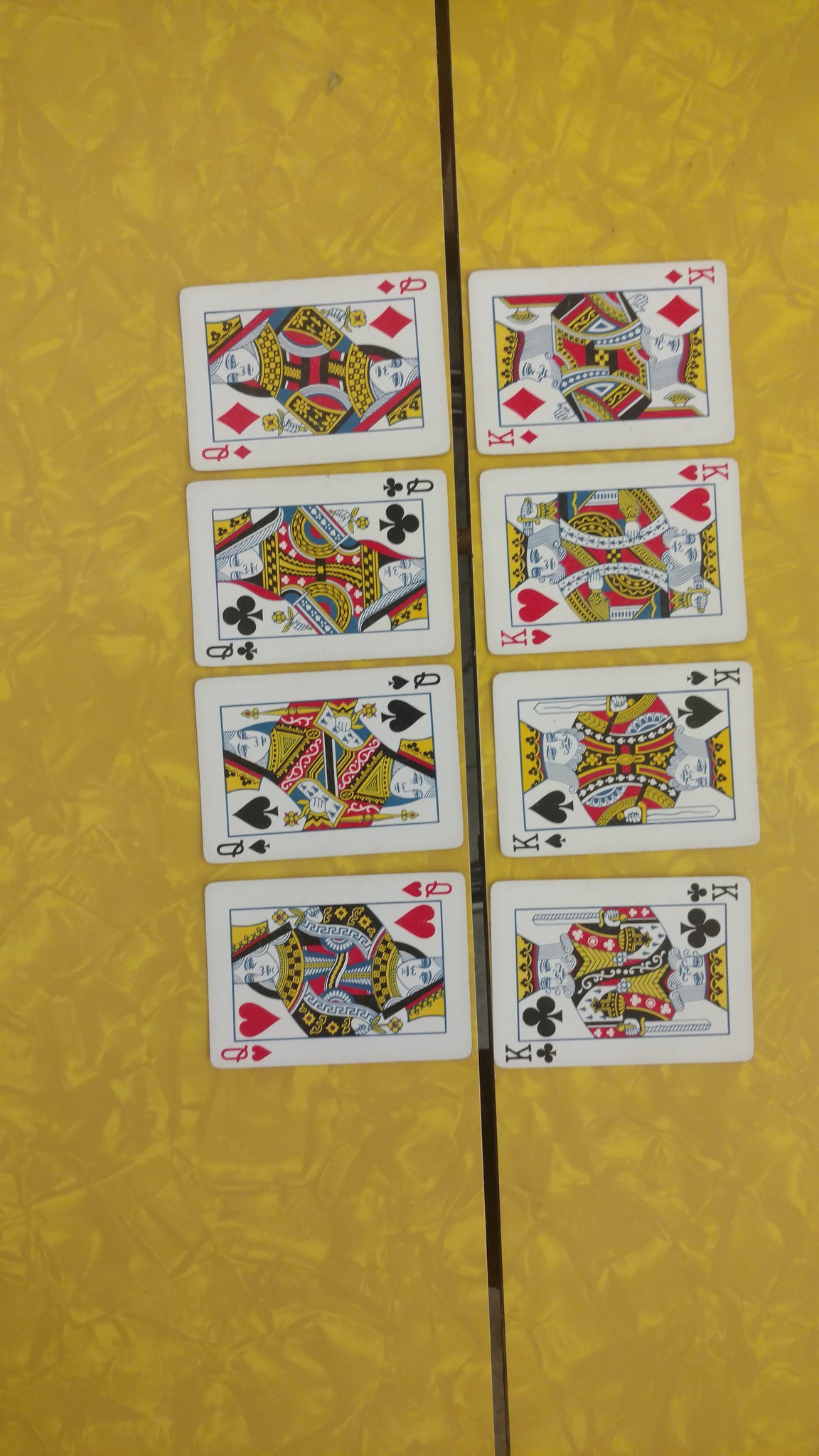The image depicts a golden yellow Formica-covered table with a grainy pattern. A dark brown line runs down the middle, marking the division between the two sections of the table leaves. On the left side of this line, four Queens from a standard American deck of playing cards are neatly lined up in a vertical column: Queen of Diamonds, Queen of Clubs, Queen of Spades, and Queen of Hearts. Similarly, on the right side, four Kings are aligned vertically: King of Diamonds, King of Hearts, King of Spades, and King of Clubs. The red suits (Diamonds and Hearts) are vividly colored, contrasting with the black suits (Clubs and Spades), which maintain their traditional shades. The cards also feature vibrant reds, yellows, and subtle blues, adding to the image's rich and detailed appearance.